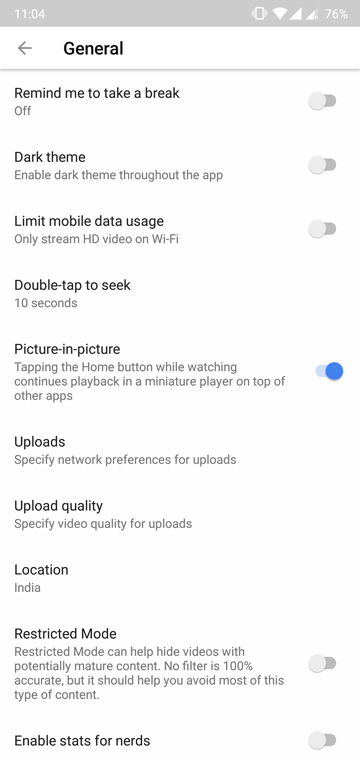A detailed screenshot from a cellphone displays various settings and options. At the top left corner, the time reads 11:04 while the icons indicate strong signal, active Wi-Fi, and a battery level at 76%. The image is focused on the "General" settings screen, which is titled at the top with a back arrow to its left.

Below the title, several options are listed:
1. "Remind me to take a break" with a toggle switch in the off position.
2. "Dark theme," described as enabling a dark theme throughout the app, also with its toggle switch in the off position.
3. "Limit mobile data usage" with a note to only stream HD videos on Wi-Fi, again with its toggle switch turned off.
4. "Double tap to seek" set to 10 seconds.
5. "Picture in picture," which mentions that tapping the home button while watching a video continues playback in a miniature player over other apps. This option has its toggle switch turned on and highlighted in blue, making it the only colored element on the screen.
6. "Uploads," where users can specify network preferences for uploading, but it lacks a toggle button.
7. "Upload quality," which allows users to specify video quality for uploads, also without a toggle button.
8. "Location" is set to India, and there’s no toggle button for this setting.
9. "Restricted mode" purports to help hide potentially mature content, with a warning that no filter is 100% accurate. This toggle switch is turned off.
10. "Enable stats for nerds," another setting with the toggle switch in the off position.

The screenshot appears to be taken from a non-iPhone device, likely a Samsung, given the layout and design of the interface. The overall aesthetic is clean, with emphasis on textual information and grayscale toggle switches except for the one blue toggle indicating the active "Picture in picture" feature.